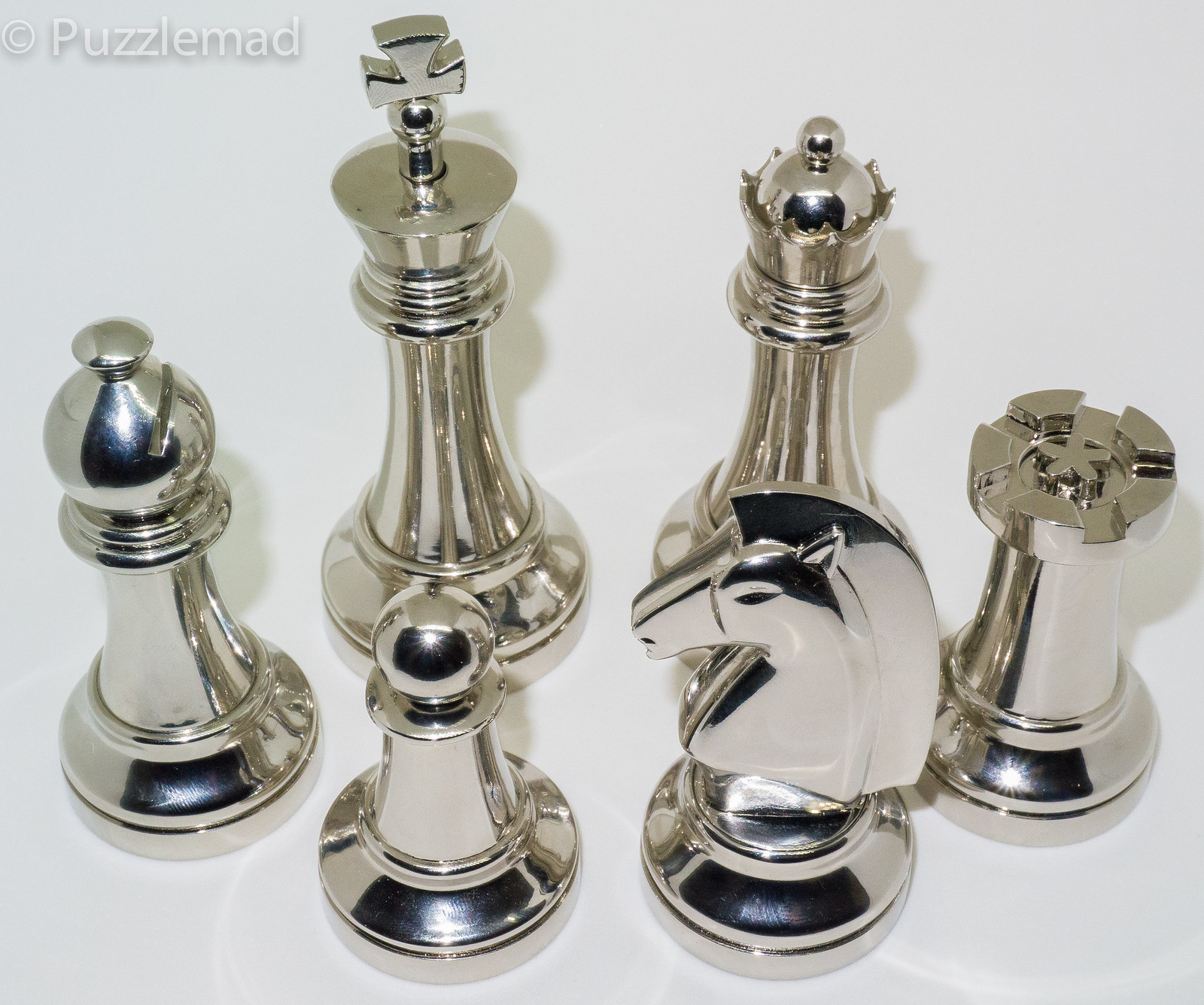This is a meticulously captured professional photograph showcasing an assortment of highly polished, ornate silver chrome chess pieces against a pristine white background that appears to be a white table. In the composition, we observe the full set of key chess figures: the king with a crown and an additional cross, a crowned queen topped with a ball, an ornate knight, a bishop positioned on the left, a rook or castle on the right, and a pawn placed in front of the king. Each piece exudes elegance with clean, modern lines. In the upper left corner of the image, there is a watermark reading "PuzzleMad" with a circled 'C', indicating copyright. The overall clarity and precision of the image suggest it is intended for professional product display.